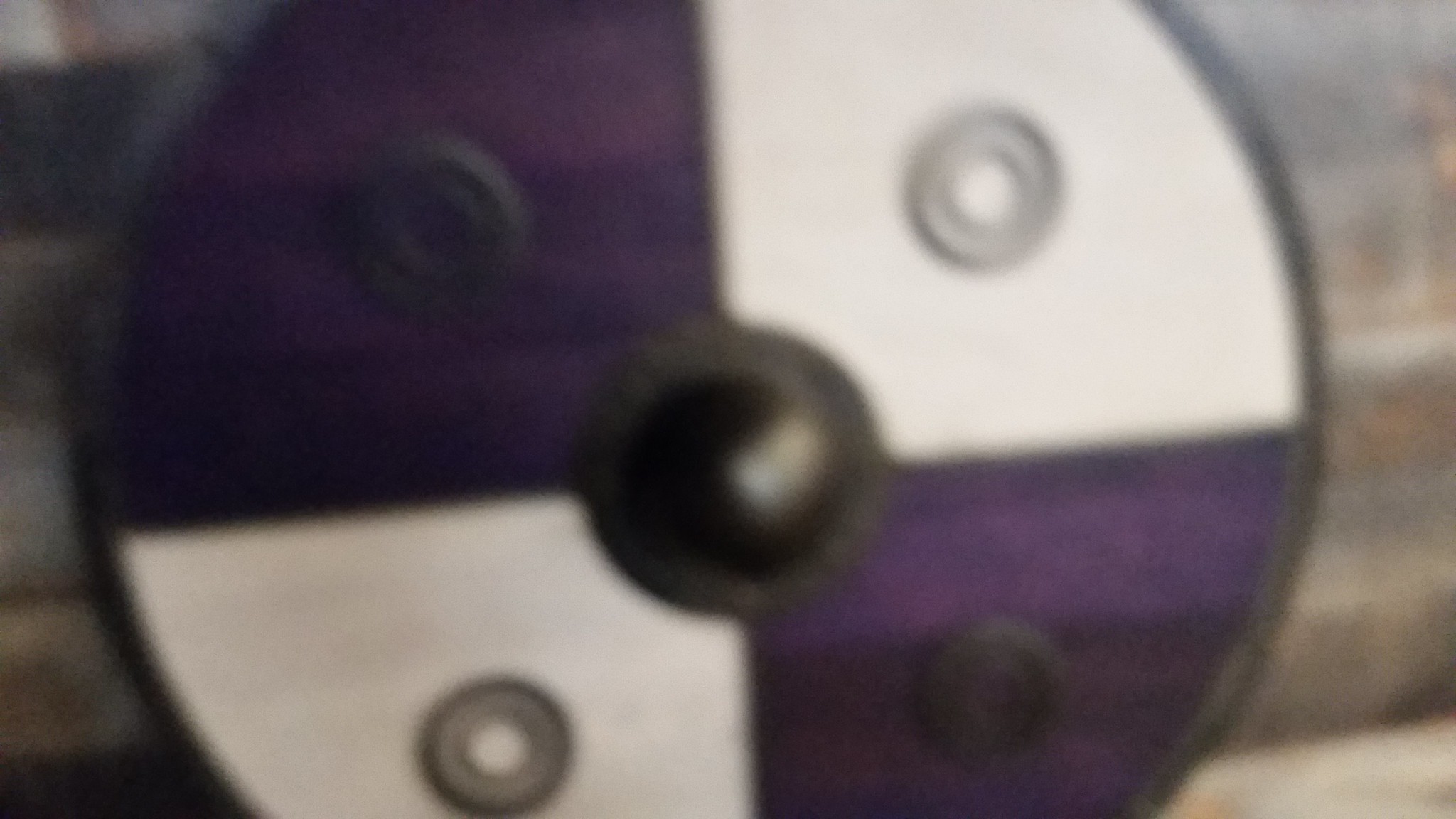The photograph features a circular object that closely resembles a medieval-style shield, akin to one you might encounter at a Renaissance fair. It is characterized by a distinct black border encircling the edge and a black center. The shield is divided into four sections: two are purple and two are white. Each white section contains a smaller white circle at its center, while each purple section features a smaller black circle at its center. The background behind the shield has a wood-grained texture, displaying varied shades of faint orange, white, and light brown, suggesting it is mounted on a wooden surface. The photo is taken in a close-up shot, resulting in a slightly grainy and blurry appearance. There are no additional elements present in the image.